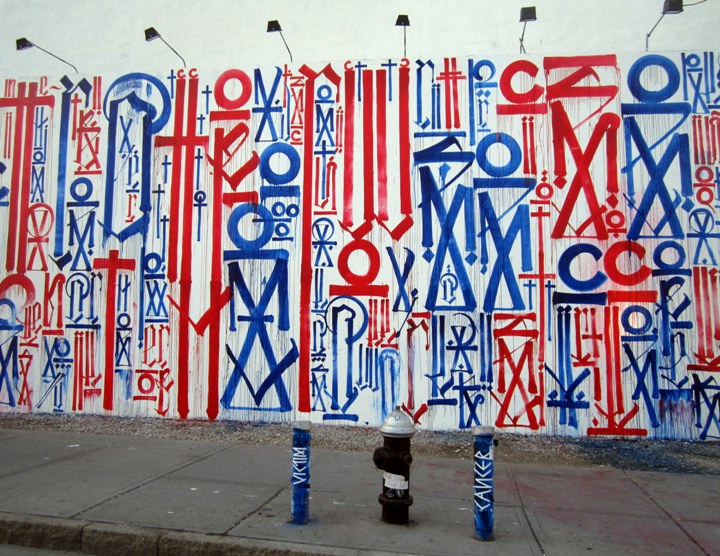The image is a photograph taken on a street featuring a detailed urban scene. The dark pavement hosts a black fire hydrant crowned with a silver cap, flanked by two short blue poles bearing white text in a foreign language. The foreground is a concrete sidewalk stained with traces of purple paint, transitioning to a strip of dead grass that has hints of blue paint scattered across it. In the background, a white wall adorned with graffiti dominates the scene. The graffiti, vibrant in red and blue, depicts various shapes including crosses, circles, M's, X's, and stick figures, interspersed with gender symbols and other abstract designs. Six black lamplights hang above the wall, casting light on this eclectic urban artwork.